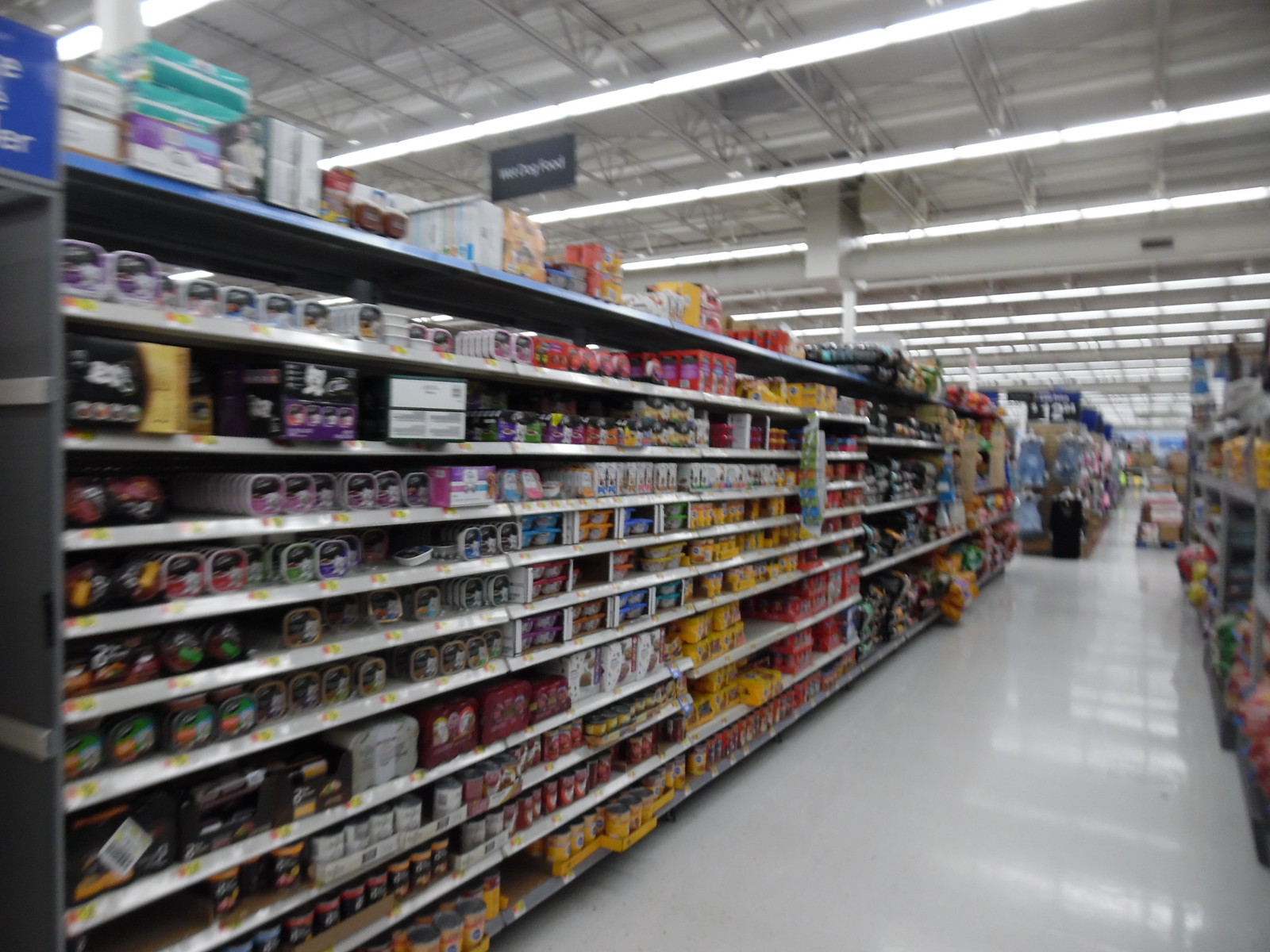In this detailed image from a pet food aisle in a grocery store, we are gazing down a well-stocked lane with shelves on both sides filled with various dog food products. The scene captures rows and rows of canned and packaged dog food, meticulously organized. On the very first top shelf to the left, a small black sign reads "dog food," introducing an array of products beneath it. Dominating the left side is the Caesar brand, with its distinctive black boxes showcasing a small white terrier on the label. Each package features the terrier against different colored backgrounds, signaling the variety within the brand. As the aisle extends, the Beneful products come into view with vibrant lids in colors like yellow, blue, pink, purple, orange, and green. Continuing further to the right, the Pedigree brand stands out with its bright yellow cans, accompanied below by the red cans of Alpo dog food. Beyond these are larger bags of dog food, adding to the assortment available.

The lane is brightly illuminated by horizontal fluorescent lights mounted on a ceiling supported by visible metal bars. The ground is a clean, stark white, reflecting the organized and tidy nature of the store. Two black signs hang from the ceiling, one positioned centrally towards the left and the other to the right, contributing to the clear navigation within the store. The overall ambiance is one of a well-maintained and thoughtfully arranged shopping environment dedicated to pet care.